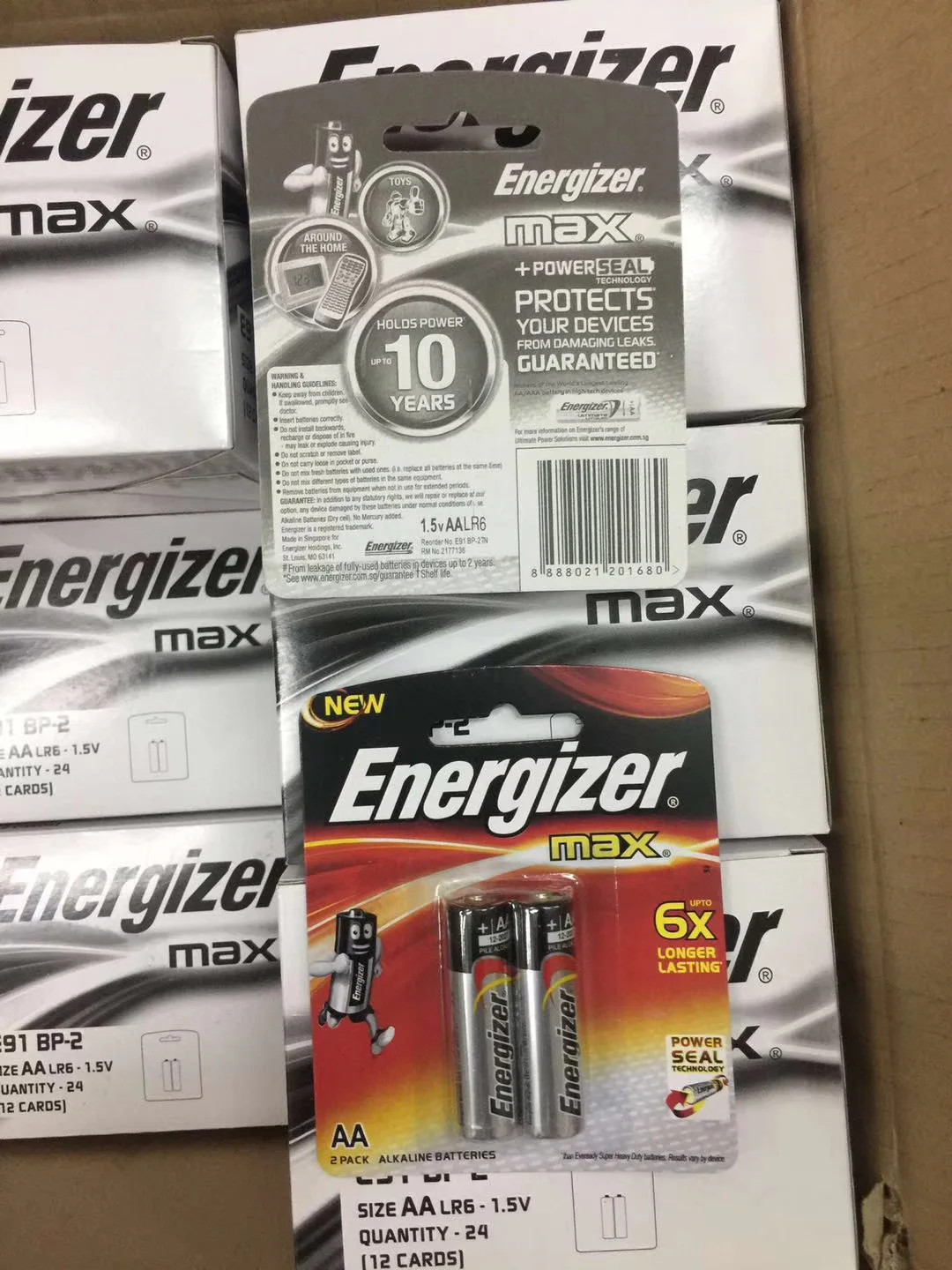The image features a textured brown surface that predominantly frames the bottom left and right sides, with a small section extending to the top left. At the bottom right of this surface, there is a hole, suggesting it might be a cardboard box. Across this surface, various packs of batteries are displayed. 

In the top left corner, a gray box is visible, likely containing some type of battery. Beneath it are two more gray boxes labeled "Energizer Max." On the right side are three additional boxes, each turned to reveal their back sides. Atop these boxes are two small packs of Energizer Max AA batteries. The topmost pack is upside down, while the pack beneath it is right side up, displaying the text and batteries clearly.